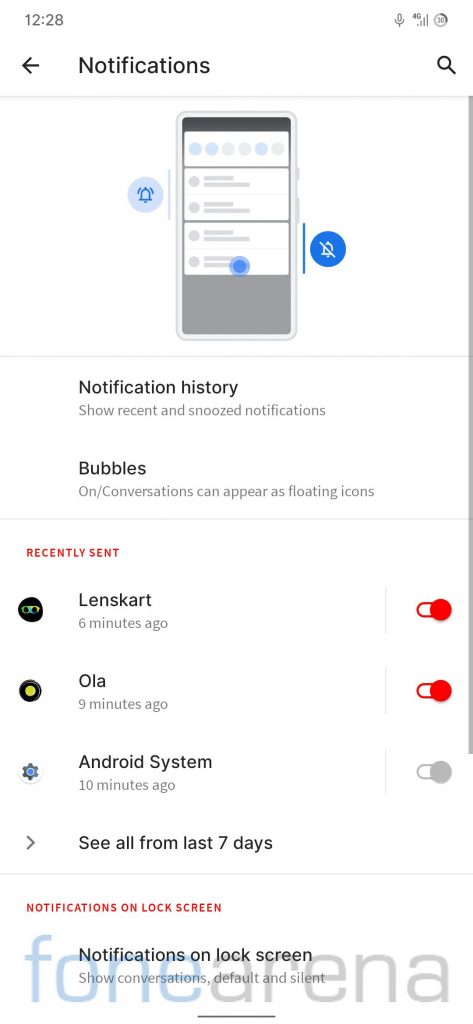The image displays a smartphone screen showing a notification management interface. At the top left, the time reads 12:28 PM, while various icons are located in the top right corner. Below, there's a search bar where users can input text. The background color is white, but the phone's display appears grayed out, with only faint colors visible at the top, including light blue, very light blue, and a yellowish tint in circular shapes.

In the primary section of the screen, bold black text reads "Notifications," accompanied by a leftward arrow. A prominent light blue circle with a bell icon indicates the general notifications section. Adjacent to this, a dark blue circle with a bell icon crossed by a diagonal line signifies the option to silence notifications.

Further down, the "Notification History" section includes a subsection titled "Bubbles" and a chronological list under "Recently sent." The recent notifications are:
- Lenskark, six minutes ago, represented by a red circular icon with a handle.
- Olga's, nine minutes ago, also indicated by a red circular icon with a handle.
- Android System, ten minutes ago, shown with a grayed-out circular icon with a handle.

At the bottom of the screen, "See all from the last 7 days" with a rightward arrow offers extended viewing of past notifications. Below that, the "Notifications on lock screen" heading appears in red text, emphasizing its importance. The background subtly displays an overlay text "Phone Arena" beneath the primary interface elements.